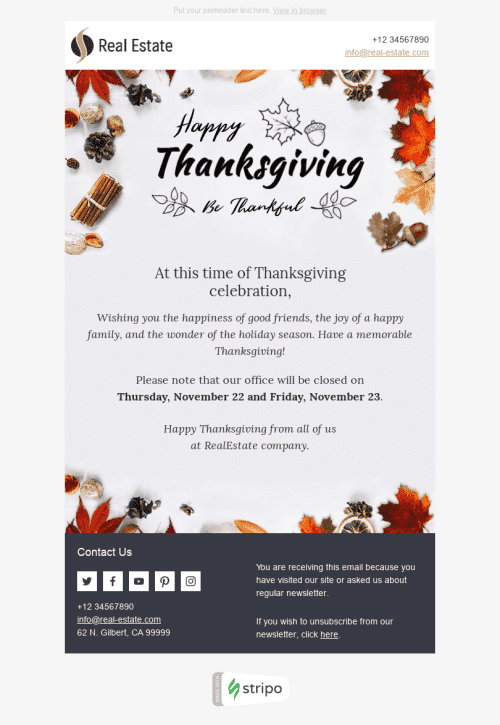The image features a light gray border encompassing all four sides. At the bottom inside this border, there is a white icon with a green symbol, accompanied by the word "Stripo" in black text. Above this is a screenshot with a white top border, featuring a "Real Estate" logo on the left side. 

The main section of the image has a slightly darker gray background than the border. It is decorated with an array of autumn elements, including fall leaves, acorns or chestnuts, cinnamon sticks, Japanese maple leaves, and star anise, evoking the scents and sights of the season.

Centered within this festive autumn arrangement is the message: 
"Happy Thanksgiving! Be thankful." Below this, a heartfelt greeting reads:
"At this time of Thanksgiving celebration, wishing you the happiness of good friends, the joy of a happy family, and the wonder of the holiday season. Have a memorable Thanksgiving."